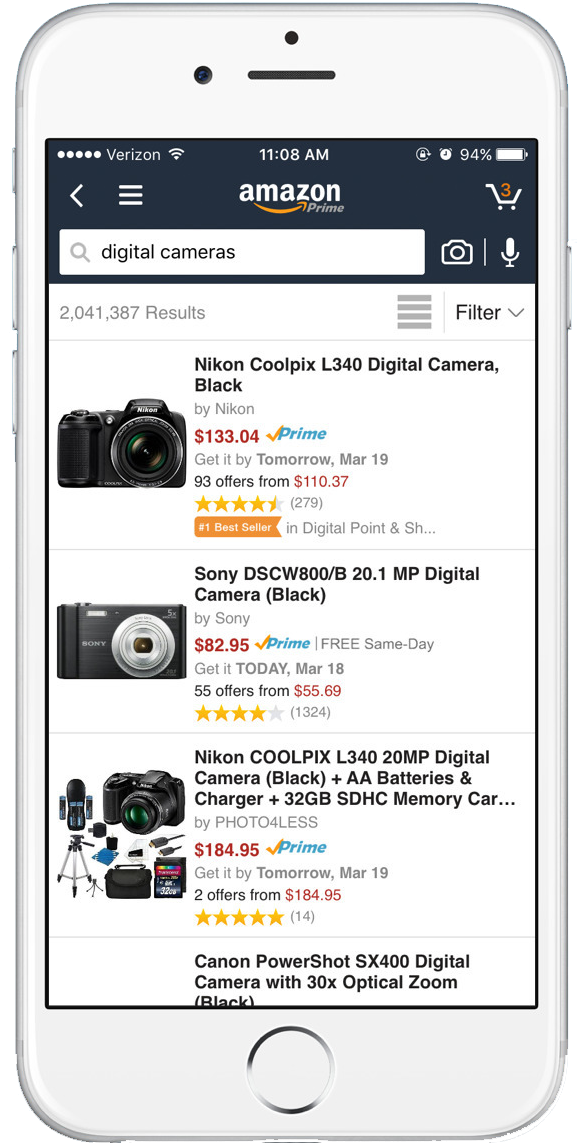The image showcases a white iPhone, partially encased in a white case, revealing its top, bottom, and right-hand side. The iPhone features a round home button with a silver ring at the bottom of the screen. On the top-left of the device, a pinhole for the camera is visible, accompanied by a small speaker grille to the right and a circular sensor above the speaker.

On the left-hand side of the iPhone, there are two volume buttons, while a lock screen button is positioned on the right. The iPhone is displaying the Amazon web page and is clearly operating on an older iOS version, identifiable by the obsolete signal indicator of five round dots on the top-left of the screen, next to the carrier name "Verizon". To the right, there are three Wi-Fi bars, the time displayed as 11:08 a.m., a screen rotation lock icon, an alarm clock icon, and the battery percentage at 94%.

Below this status bar, there is a white left arrow, three horizontal lines, and the Amazon logo indicating Amazon Prime. The cart icon, featuring the number three, is positioned to the right. Below these icons lies a search bar with a magnifying glass symbol, and the query typed in lowercase letters: "digital cameras". Additional icons for camera and microphone are placed to the right of the search bar.

The results section of the Amazon page, set against a white background, lists 2,041,387 results with filters on the right. The first listing is for a Nikon Coolpix L340 digital camera (black) priced at $132.04, available on Amazon Prime with delivery by tomorrow, March 19th. It boasts 279 reviews with an average rating of four and a half stars. The listing includes an image of the black camera.

The second listing features the Sony DC-W800-B 20.1MP digital camera (black), priced at $82.95, also available on Amazon Prime with same-day delivery. It has 1,324 reviews with four stars and an image showing the black camera with a silver lens.

The third listing, a Nikon Coolpix L340-20MP digital camera (black) package from Photo4Less includes AA batteries, a charger, and a 32GB SDHC memory card, priced at $184.95, available on Amazon Prime with delivery by tomorrow. It has five stars from 14 reviews and comes with additional features like a tripod, memory card, case, and cables, visible in the image.

The final listing that is partially shown is a Canon PowerShot S6400 digital camera with 30x optical zoom (black).

This detailed description covers the visual and textual elements displayed on the iPhone screen, highlighting the specific features of the device and the content of the Amazon web page.